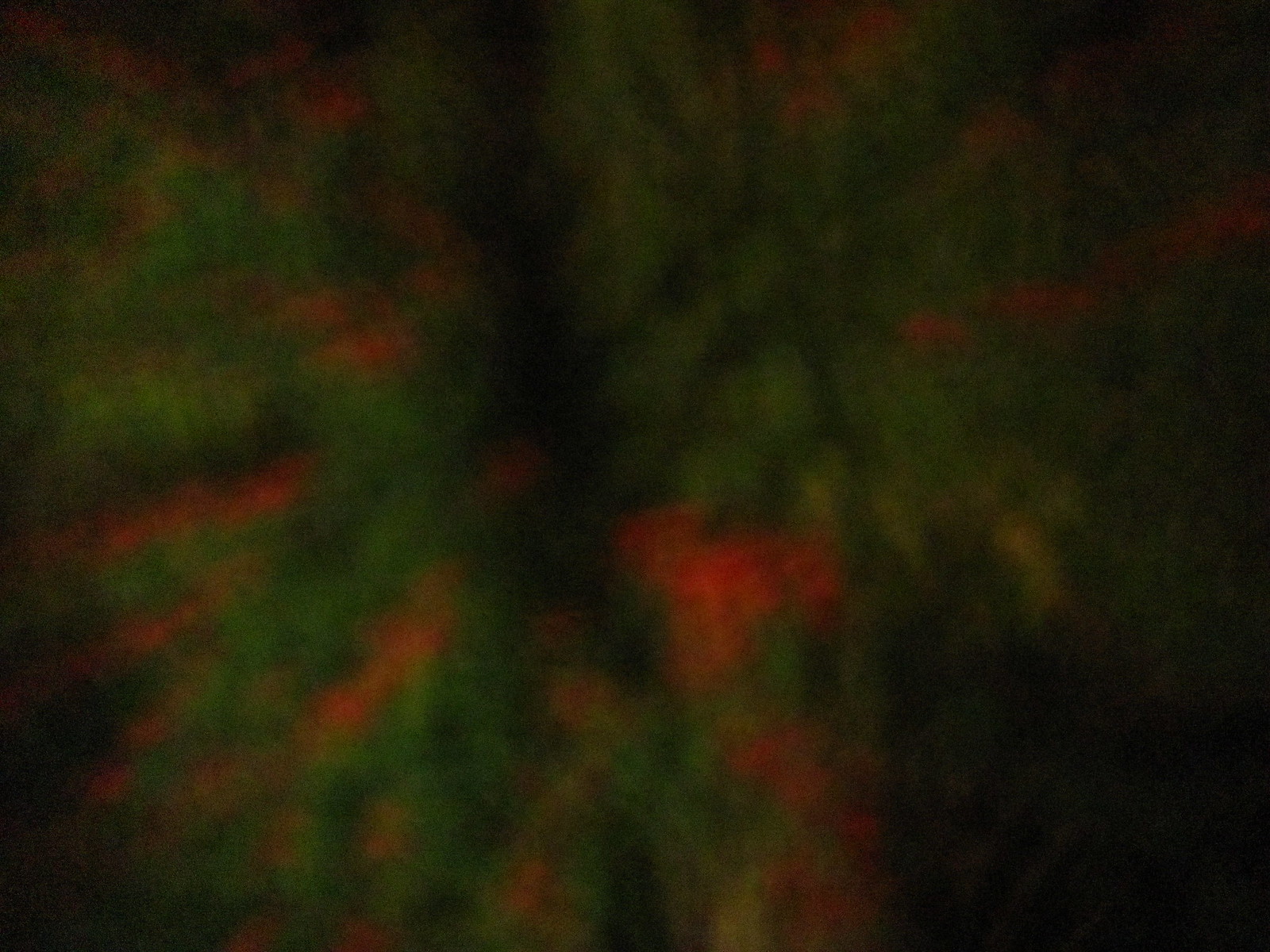This image is highly blurred, making it difficult to discern precise details. However, it predominantly features dark green circular objects adorned with red accents––likely Christmas wreaths decorated with bright red bows. These wreaths appear to be stacked atop one another, creating a layered effect. The green and red items form a circular pattern around the photo's center, with one extending towards the upper right corner. The photograph itself has blackened corners, adding to its obscure nature. Additionally, some of these green circular items with red bows are also situated at the bottom of the image, reinforcing the impression of festive, evergreen wreaths.